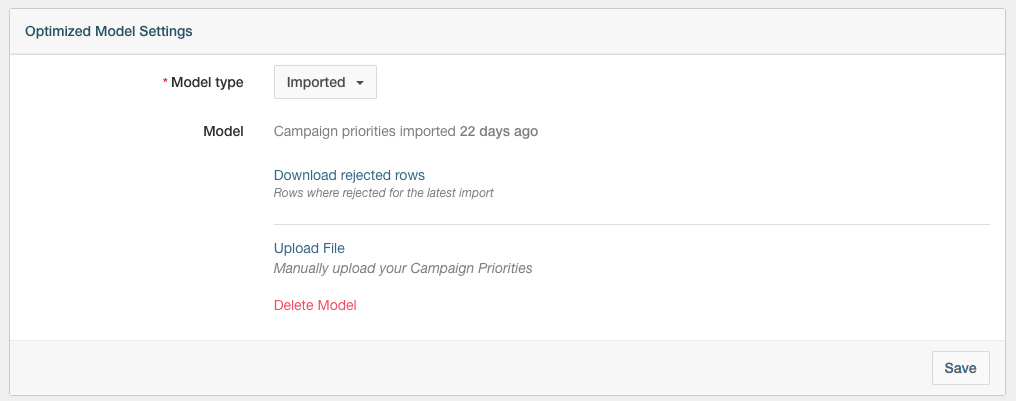A detailed visual representation of the "Optimize Model Settings" window is prominently displayed in this image. The window, positioned in the top left-hand corner of the screen, is primarily white in color, providing a clean, minimalistic interface.

At the top, the window bears the title "Optimize Model Settings," indicating its purpose. Beneath this header, the main section of the window is divided into two columns.

On the left, there is a label that reads "Model Type," and to its right, the word "Imported" is displayed, signifying the nature of the model being utilized. Directly below, the label "Model" is followed by a descriptive note specifying that the campaign priorities were "Imported 22 days ago."

Further down, the window states "Download Rejected Rows," explaining that the rows were rejected during the latest import process. Immediately beneath this, there is an option titled "Upload File Manually," inviting users to manually upload their campaign priorities.

At the bottom of the window, there is a notable red-font option labeled "Delete Module," presumably for removing the module entirely. To the far bottom right, a small rectangular button with the word "Save" on it provides the option to preserve any changes made within this window.

Overall, the visual interface clearly delineates options to optimize settings, manage uploads, handle rejected rows, and save or delete the module.